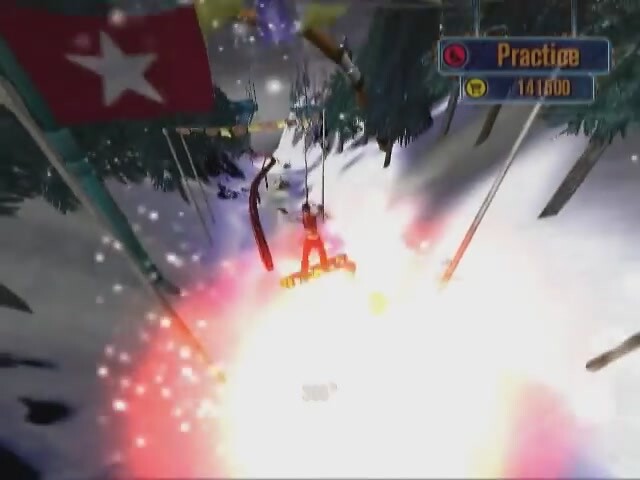This vibrant rectangular image appears to be a photograph taken from an elevated perspective, although it is somewhat overexposed, adding to the bright, ethereal quality of the scene. Prominently displayed is a red flag adorned with a single white star, mounted on what appears to be a green pole. To the right, two distinct signs are visible: one reads "Practice" and another displays "14 1 500." The background suggests a ski resort setting, featuring glimpses of trees amidst the brightness. However, the image seems to be a composite, merging elements from different sources to create an eye-catching, sparkling effect, replete with abundant whites and other stark highlights. This artistic combination imbues the photo with a sense of whimsy and fantasy, transcending the ordinary and inviting viewers to look closer.